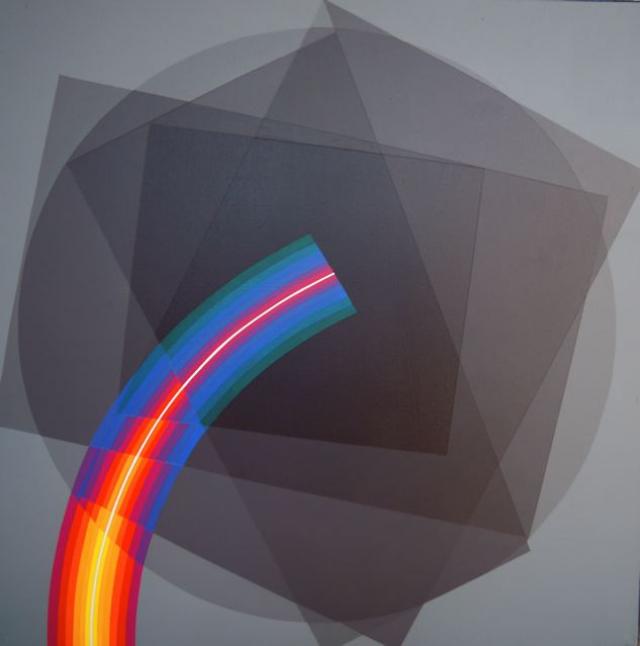This digital artwork features a light gray background with a collection of overlapping geometric shapes rendered in varying shades of gray. These shapes, including rectangles, squares, triangles, and a circle, become darker where they intersect, creating a sense of depth and complexity. Dominating the composition is a multicolored, ribbon-like object that begins near the bottom right corner, arches gracefully toward the center, and then extends downward to the bottom left of the image. The ribbon transitions in color from bright yellows, oranges, reds, and purples at its base to blues and dull greens as it progresses upwards. A bright white line runs through the vibrant colors, adding an electric, dynamic touch. This intricate design, approximately eight inches by eight inches, lacks any visible signature or textual elements, focusing solely on its striking visual interplay of shapes and vibrant hues.